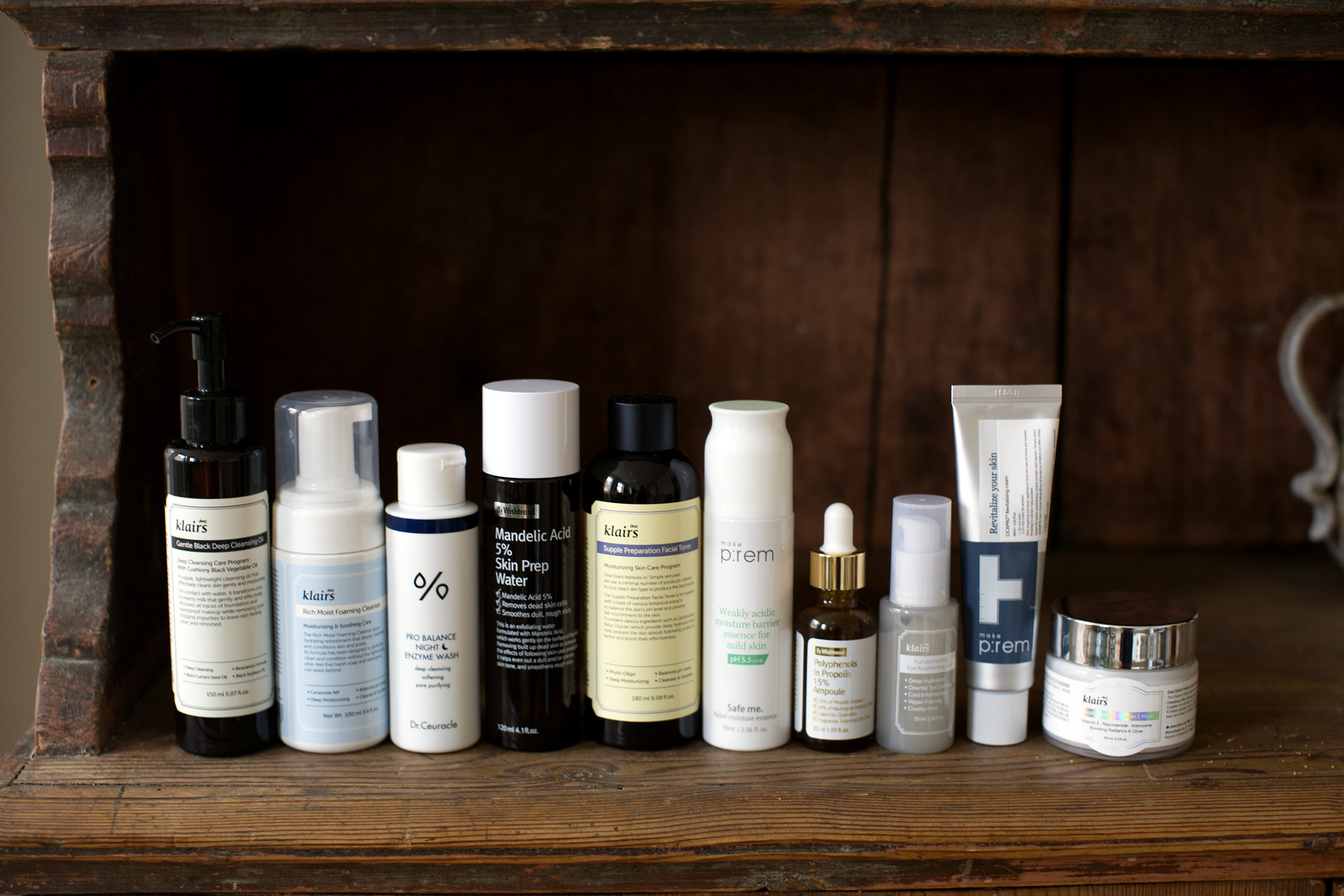A detailed image caption could be:

"A neatly organized wooden shelf, possibly serving as a tabletop, holds an array of skincare products against a beige wall. There are ten items meticulously lined up from left to right. Starting from the left, the first item is a black pump bottle with a white label that reads 'Klairs Gentle Black Deep Cleansing Kit,' featuring various ingredients listed below. The second item is another product from Klairs, a 'Rich Moist Foaming Cleanser,' with its ingredient list visible. 

The third item stands out with a logo design resembling teardrops or a percentage symbol, labeled 'Pro-Balance Night Enzyme Wash' from Dr. Ceuracle. Next is a sleek black bottle with a white cap, reading 'Mandelic Acid 5% Skin Prep Water,' accompanied by a list of ingredients.

Following this is yet another Klairs product, which appears to be a facial toner, although the text is hard to read. The sixth item is a white bottle labeled 'Prem Weekly Acidic Barrier' for mild skin. Near the center is a small serum bottle with text indicating it contains 15% of an unspecified ingredient. The eighth item is a smaller pump bottle from Klairs with an unreadable label.

Next, there’s a silver tube with a white cap, labeled 'Prem Revitalize Your Skin,' stored upside-down on its cap. The final item to the right is another Klairs product, presented in a glass jar with a tin silver top. Adjacent to the collection, a shiny silver handle, possibly of a pitcher, peeks into the frame from the right side."